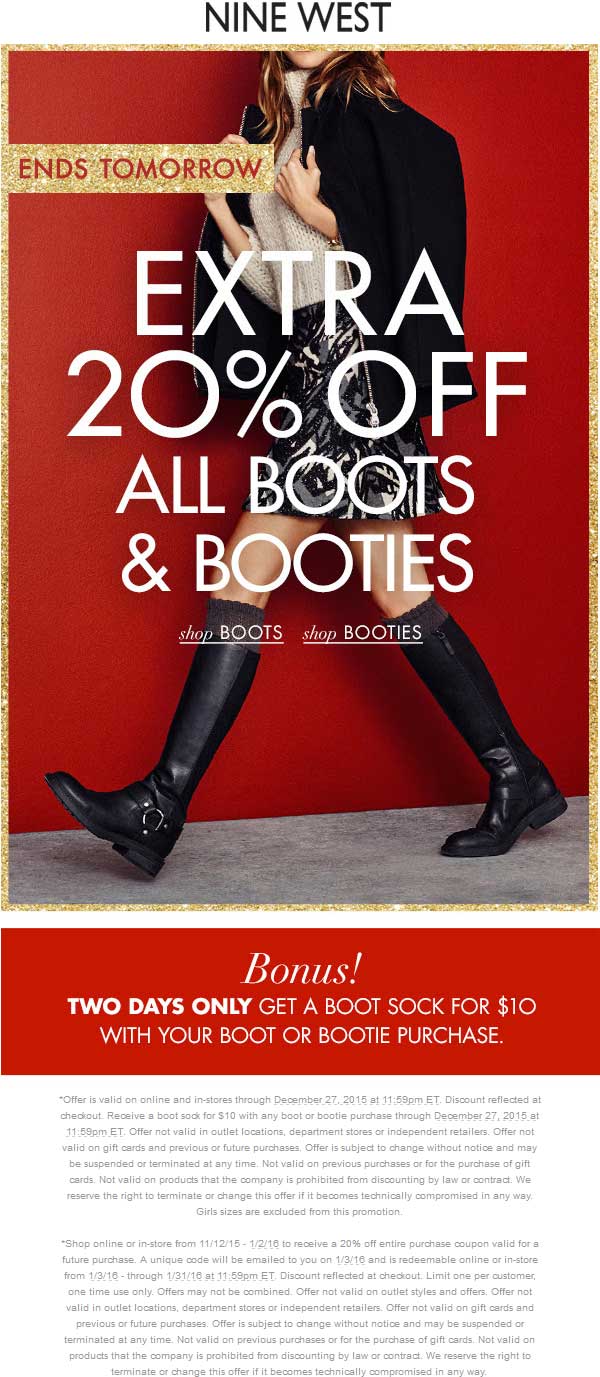The color advertisement for Nine West features a stylish woman confidently walking. She is adorned in chic black leather knee-high boots that complement her sophisticated ensemble. Her outfit includes a sleek black coat with a zip-up front, paired with a multi-colored skirt in shades of gray, black, and white. She completes her look with a light-colored sweater. The background is a striking red, drawing attention to her polished appearance. 

Superimposed on the image, in bold white text, is an enticing offer: "Extra 20% off all boots and booties." Above this, a smaller banner indicates urgency with the phrase "Ends Tomorrow." Directly beneath the woman, a prominent red banner highlights a "Two Day Bonus," and the bottom of the image features fine print details in grayish text on a white backdrop. This meticulously crafted advertisement is eye-catching and urges viewers to take advantage of the limited-time deals at Nine West.